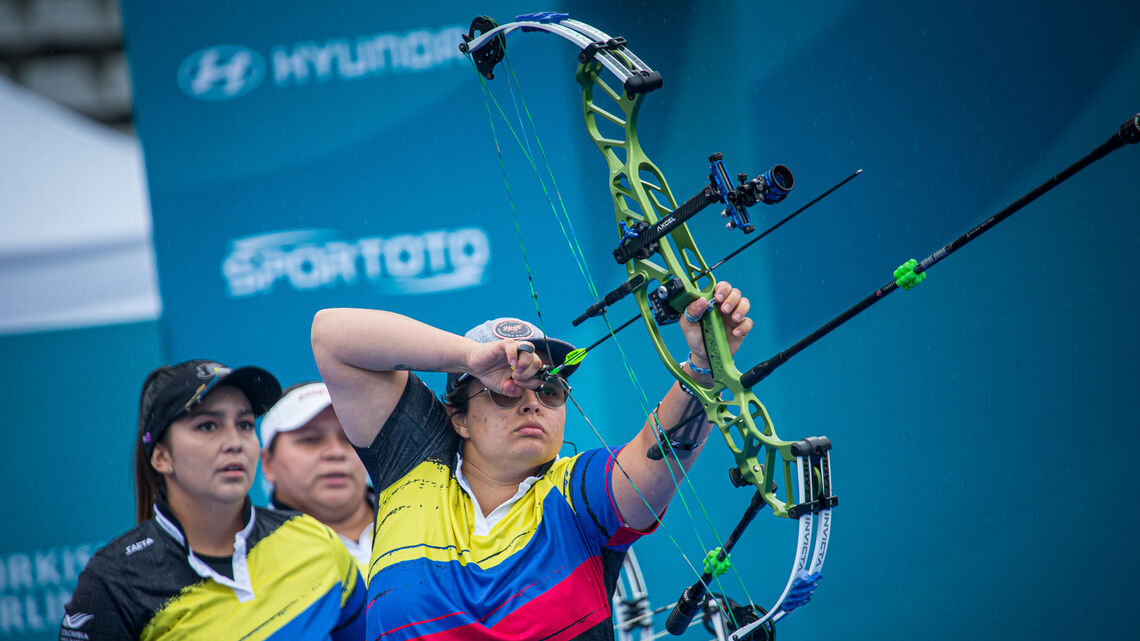In the image, an archer, possibly of Colombian or Venezuelan descent, is seen preparing to draw and shoot a neon green compound bow equipped with tactical accessories, including a scope and counterweights. The archer is wearing a white baseball cap with blue trim and sunglasses, coupled with a black, yellow, blue, and red striped polo shirt, which seems to be part of a team uniform. Beside and behind the archer are two teammates also in the same striped shirts; one has a black baseball cap with a visible ponytail, and the other is mostly obscured, wearing a white cap. The archer is also equipped with essential archery gear such as a finger tab or trigger and a wrist guard to mitigate the impact of the bowstring. Logos in the blurry background include "Sportoto" on a bright blue wall, likely representing sponsorships or event associations, alongside a visible "Hyundai" logo. The archery scene is heightened with the archer nocking an arrow, poised to take a precise shot.